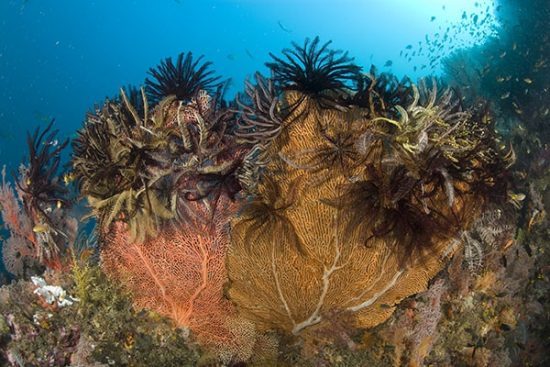The underwater photograph captures a mesmerizing aquatic scene with a distinct rectangular shape, where the top and bottom sides are twice as long as the left and right sides. The entire image is suffused with a bluish tinge due to the water, which imparts a serene blue filter across the scene. In the top left corner, the water stretches into the distance, creating a tranquil horizon that transitions from a lighter blue on the right to a darker blue towards the top right corner.

Dominating the photograph is a vibrant display of underwater plant life. Prominent are the coral and frond-like plants that take up much of the space, resembling ferns with multiple small stems adorned with frilly, leaf-like fixtures in shades of black and yellow. These delicate fronds sit atop larger, stony-looking formations in orange and yellow hues, contrasting with the softer plant textures.

Adding to the complexity of the scene, the background features a gentle slope of rock and soil debris under the water, while the darker upper right corner hints at depth. Scattered among the plant life, one can observe small fish drifting amidst the blue water, enhancing the dynamic and lively nature of the underwater environment. The fish, combined with the array of colors from dark green and brown to peach, tan, and gray, create a rich tapestry that highlights the diversity and beauty of marine ecosystems.